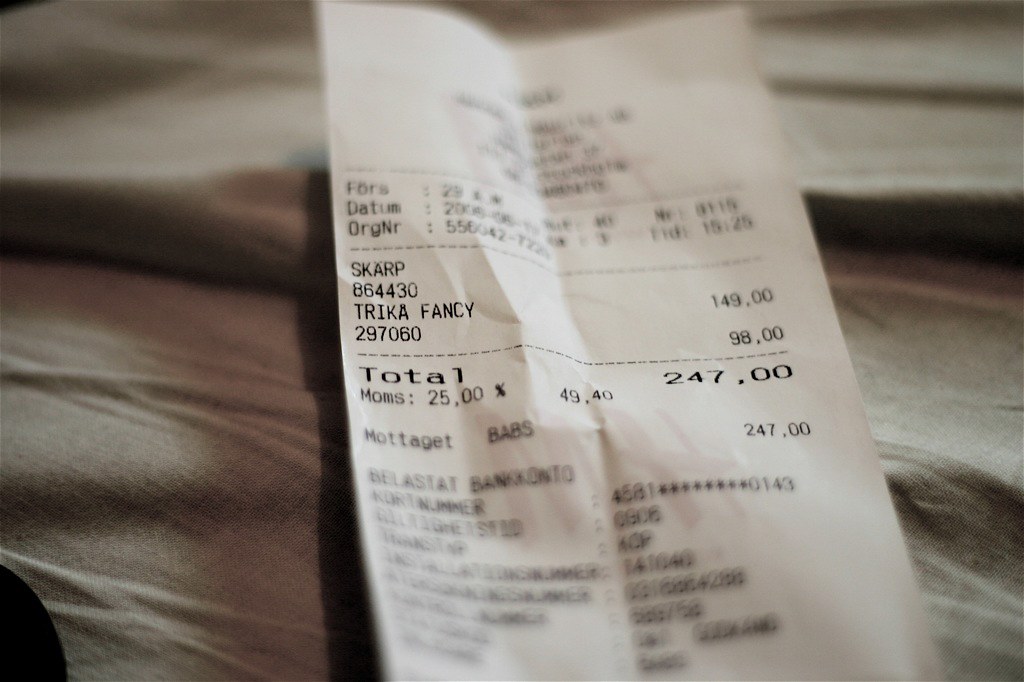This image showcases a slightly blurry, close-up photograph of a wrinkled receipt positioned on a bunched-up piece of brown, linen-like fabric. The receipt, which appears to have been folded in half vertically and then unfolded, is mainly obscured at the top and bottom. However, key details are visible in the middle section. The receipt lists "SCARP" followed by the number "864430," and below that, "TREKA FANCY" priced at "149.00" along with another item priced at "98.00," leading to a total amount of "247.00." An indiscernible, circular object is noticeable in the lower left-hand corner. Shadows cast by the receipt and surrounding fabric add depth to the dimly lit composition.